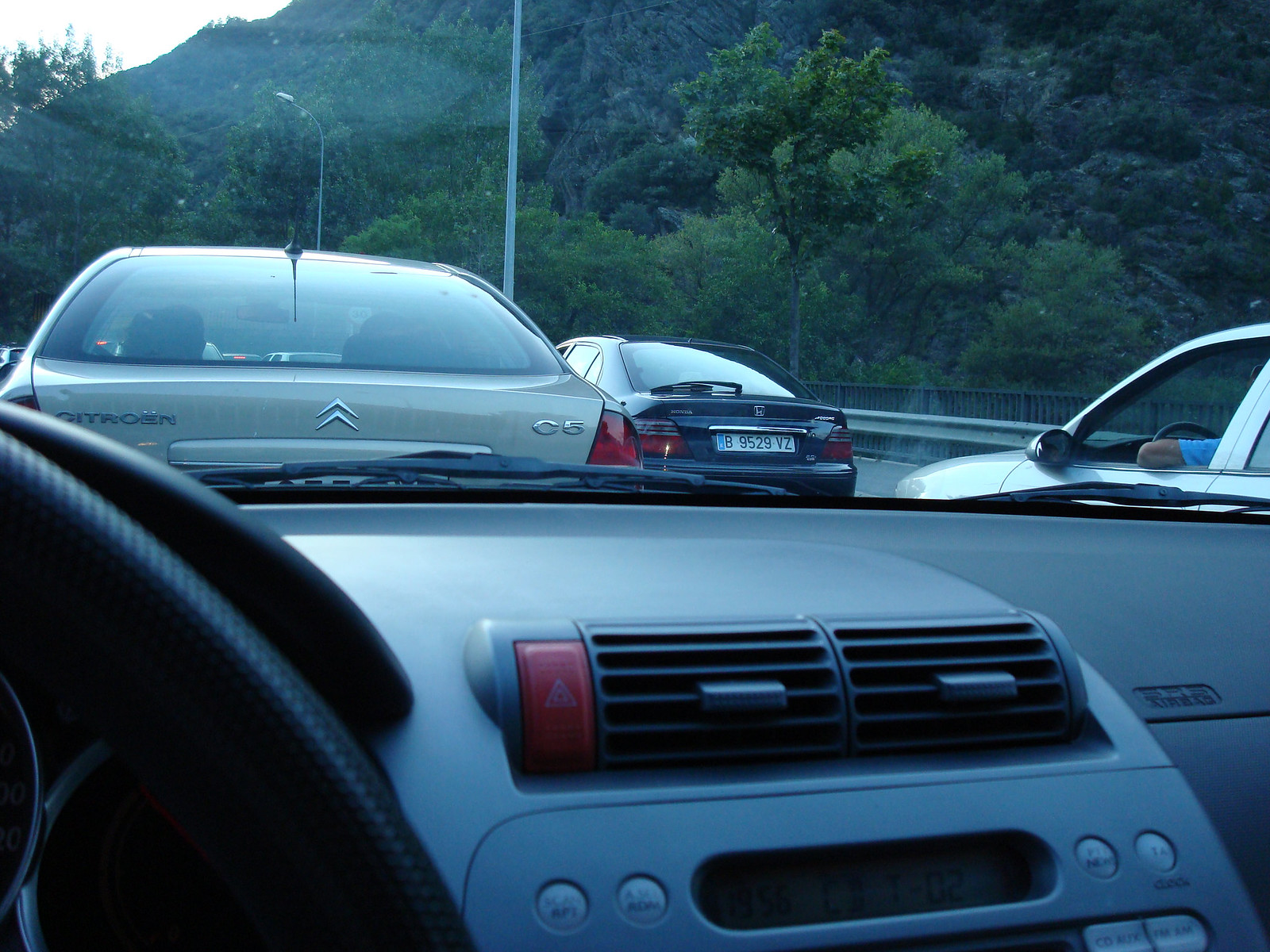This interior shot of a car captures a close-up view of the dashboard from the driver's perspective. On the left-hand side of the image, a portion of the steering wheel is visible. Centrally located are two air vents, adjacent to which is a red hazard button positioned to the left. Below the vents are four circular control buttons. To the right, a section of the black dashboard is shown. Looking out through the windshield, three cars are visible: one silver vehicle directly ahead, another silver car to the right, and a darker-colored car, possibly dark blue or black, positioned in front of the right-side silver car. In the background, a couple of light posts stand amidst a lush landscape with abundant trees and greenery, suggesting a hill rising behind the treeline. A sliver of sky can be seen in the top left-hand corner, adding depth to the scenic view outside.